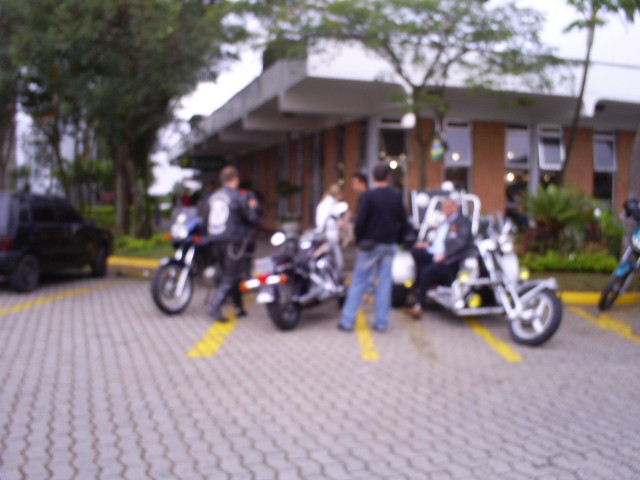The photograph depicts a daytime scene of a parking lot made of distinctive zigzag or octagonal brick tiles, not typical for usual parking lots. The blurred image shows several motorcycles, mostly black with some featuring long handles, parked in narrow spaces delineated by yellow lines that create four stalls. To the left, a black SUV is visible. Three men are near the motorcycles: one in jeans and a dark jacket, another in black pants and a leather jacket adorned with a logo, chain visible on his hip, and a third who seems to be leaning on a motorcycle. Another person in white stands in front of the building, which appears educational or administrative, with slim windows and brick walls forming an angle. Trees and greenery surround the area, especially on the left. The bright yellow curb stands out, adding to the overall impression of an overcast day in a location that doesn't resemble the smooth concrete roads commonly seen in the United States.